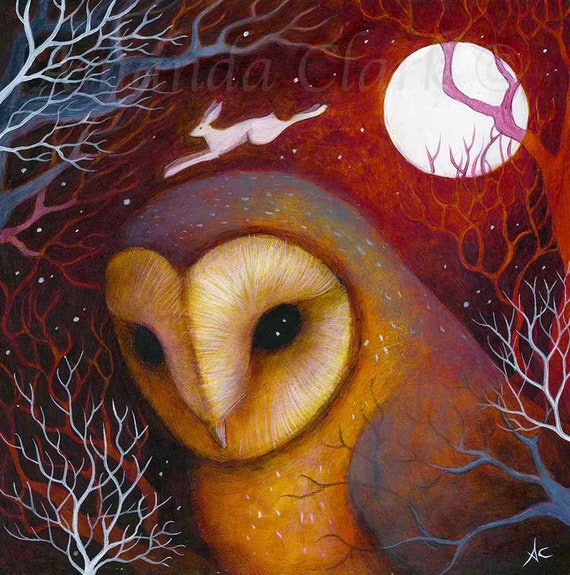The painting features a prominently displayed owl in the foreground, characterized by a white face, black eyes, and a pointy beak. The owl's body is primarily brown, with lighter tan hues on its face and chest. The background of the image is a vivid red, complemented by barren tree branches in various shades of white, red, and light pink, which frame the scene. Delicate white dots dispersed throughout the background evoke a sense of light snowfall, contributing to a wintry atmosphere. Above the owl's head, a dynamic white rabbit appears to be in mid-leap, with its front paws stretched out ahead and back legs extended behind. To the right of the rabbit, a bright, white moon illuminates the scene. Faint lettering can be discerned at the very top center of the painting, with the characters "N-D-A-C-L-A-R-C" partially visible among the darker background tones. The detailed composition and high-quality execution of the artwork make it a visually compelling illustration.